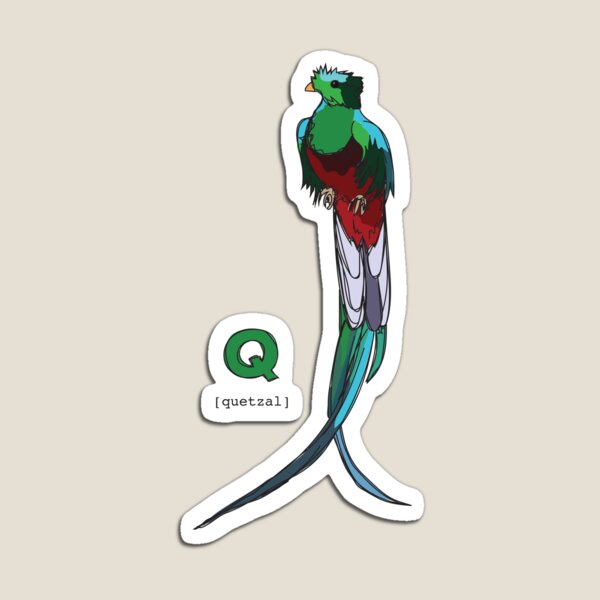The image showcases a vibrant, artistic sticker or illustration set against a muted gray-beige background. At the center of the image is a detailed depiction of a slender, majestic parrot with long tail feathers that extend to the bottom of the image. The parrot's head features a blend of green, blue, and black colors, and it has a small orange beak. The body continues the green and blue hues, while the belly is bright red. The tail feathers exhibit a mix of light purple, gray, green, and blue, giving them a striking, flowing appearance. The entire bird illustration is outlined in white, enhancing its prominence against the background. To the left of the parrot is a smaller illustration or logo featuring a large green "Q" with the word "Quetzal" underneath. The overall style of the image is artistic with a slight cartoonish flair, emphasizing both the beauty of the bird and the elegant simplicity of the surrounding elements.